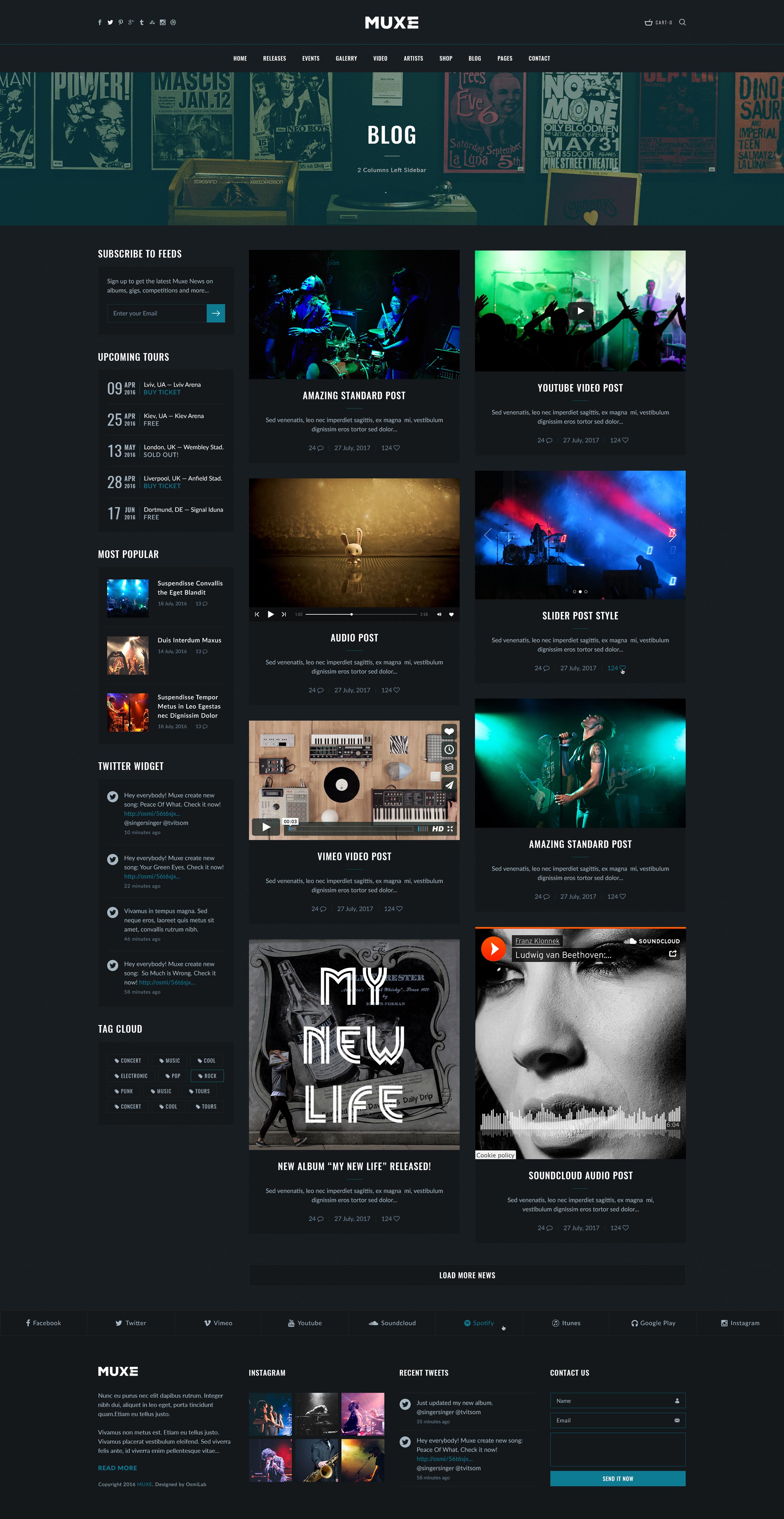**Detailed Screenshot Caption**

This image is a detailed screenshot, likely from a tablet device, displaying a multimedia platform interface. The overall background is a dark shade, either black or dark gray. At the top of the screen, there are several small icons for social media and search functionalities, including Twitter, Facebook, and Google. Centrally positioned at the top, "MUXE" is displayed in bold, white capital letters, and to the right, there's a tiny icon labeled "Cart" next to a search icon.

Beneath this header, there is a lighter-colored bar, which appears slightly translucent, containing a series of posters. There are approximately eight posters featured in this bar. The first poster shows Malcolm X, with an arm raised and pointing, under the word "Power." Another poster features the punk rock band, Neo Boys, and another announces "No More Oily Blood Men," dated May 31st. Yet another poster displays a title that includes "Dinosaur," although the complete text is partially obscured.

In front of the poster section, "BLOG" is boldly written in capital white letters, marking the beginning of the blog content area. This main section contains various media posts, including both video and audio clips, primarily featuring rock bands. Each post displays images of crowds, musicians, including singers, guitarists, and drummers. One notable post shows a toy rabbit floating in water against a sandy-colored backdrop, designated as an audio post. Another post from Vimeo features several musical instruments scattered on a wooden floor, such as organs and keyboards.

Additionally, a highlighted post presents a close-up of a woman's face with the text "Franz Klonnak" and "Ludwig van Beethoven" along with an indication that it is a SoundCloud audio post. The post includes metrics like repost count, likes, and a timestamp of July 27, 2017.

On the left-hand side, a sidebar lists various categories. The first category invites users to "Subscribe to Feeds" with a spot for entering an email address. Following this, the "Upcoming Tours" category lists events for April 2016 in London and other locations. The next section, "Most Popular," showcases three pictures with titles. Then, a "Twitter Widget" displays four posts, one beginning with "Hey everybody," referencing the creation of a new song, though some text remains unreadable due to small font size. Another section labeled "TagCloud" gathers tags for quick navigation.

At the bottom of the screen, there are several clickable tabs for different platforms, including Vimeo, YouTube, Google Play, and Spotify, with Spotify currently highlighted, indicating the page's primary focus. The footer features "MUXE" once more with additional context and links. Adjacent sections display six Instagram images and a "Recent Tweets" area with two tweets, ending with a "Contact Us" section for user inquiries.

This comprehensive interface offers a diverse range of multimedia content, interactive social features, and user engagement options, all organized within a sleek and dark-themed design.